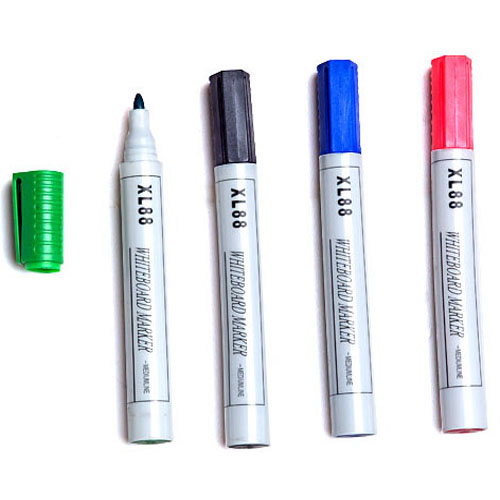This photograph features a set of four vertically oriented white dry erase markers, each with the label "XL88" and "whiteboard marker" in black text on a white background. The markers are arranged from left to right with the following cap colors: green, black, blue, and red. The cylindrical markers are identical aside from their cap colors, which also match the bottoms of each marker. The green marker on the far left has its cap removed and placed beside it, revealing its green felt tip. The background of the image is white, providing a clean and contrasting backdrop that highlights the colors and details of the markers.